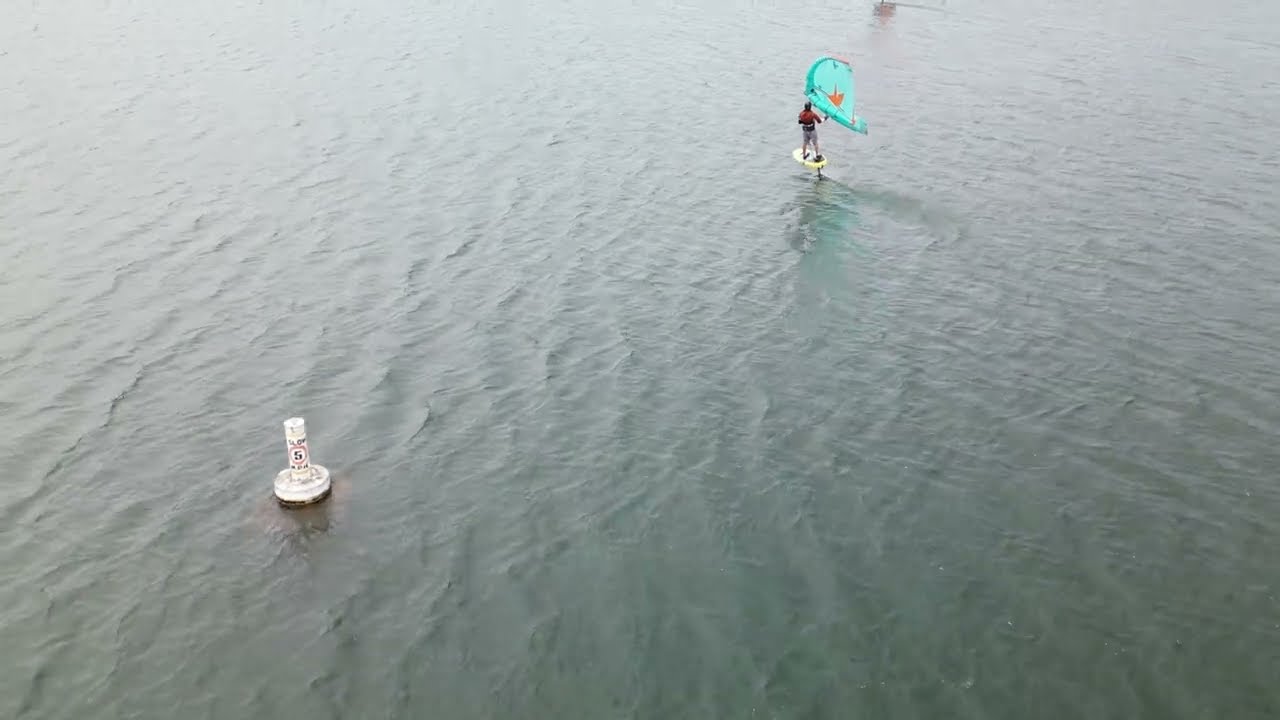The image captures a calm, expansive body of greenish-gray water, filling the entire frame. In the lower left corner, a white buoy floats, marked with the number "5" in black and encircled by red. Toward the upper right, a man in a red shirt and gray shorts stands on a small, white paddleboard. He grips a turquoise blue sail, adorned with what seems to be an orange star or leaf, likely indicating he's windsurfing. The serene outdoor setting—possibly a lake or ocean—is devoid of any text, adding a pure, uninterrupted view of this aquatic scene.